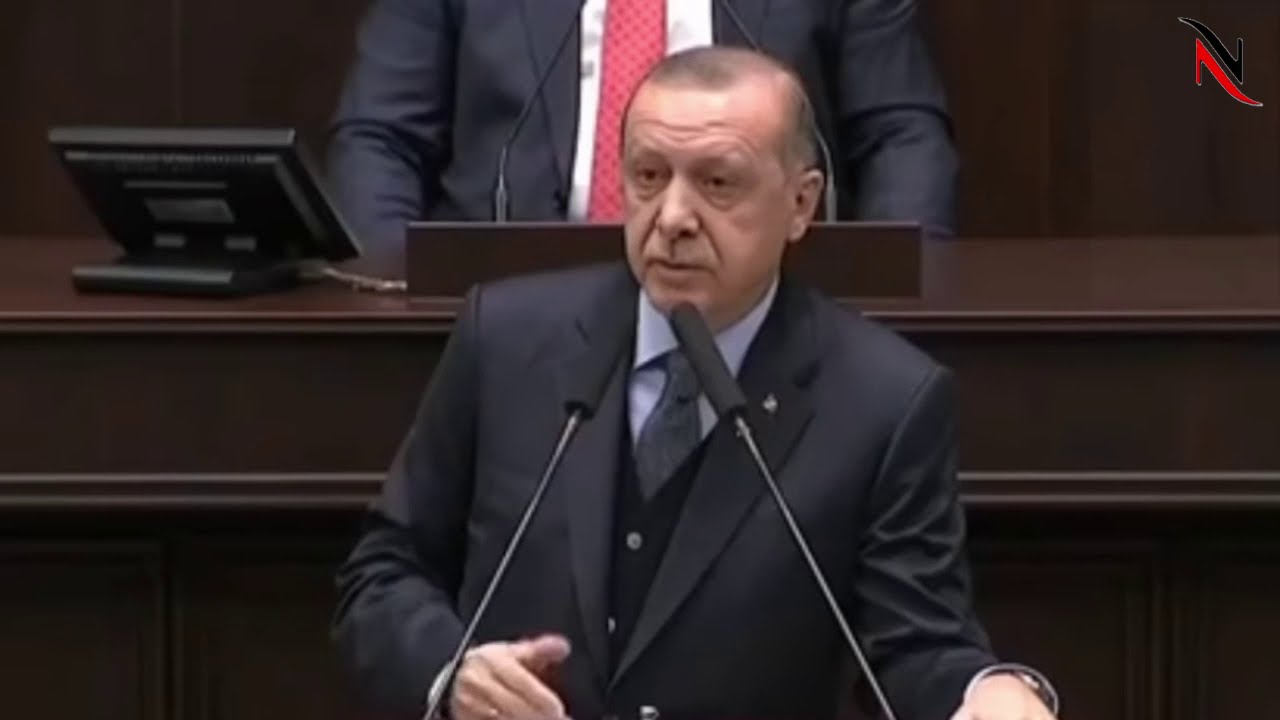In the foreground of the image, an elderly white gentleman with minimal hair stands at a podium, although the podium itself is not visible. Flanking his face are two long microphones, one positioned to the left and the other to the right. He is dressed in an elegant ensemble consisting of a black suit jacket, a dark black vest, a gray tie, and a white shirt. Partial views of a ring on one hand and a watch on the other are evident. 

Behind him, there is a raised wooden seating section characterized by its dark brown hue and a mix of outlined rectangular doors at the bottom and a smooth, flat surface at the top. A seated individual, adorned in a black suit with an open jacket, a white shirt, and a red polka dot tie, is visible with an open computer in front of him on the left. Two microphones extend from the console in front of the seated man. The setting appears to be a formal environment, possibly a court hearing or a political assembly, indicated by the formal attire and the layout of the surroundings.